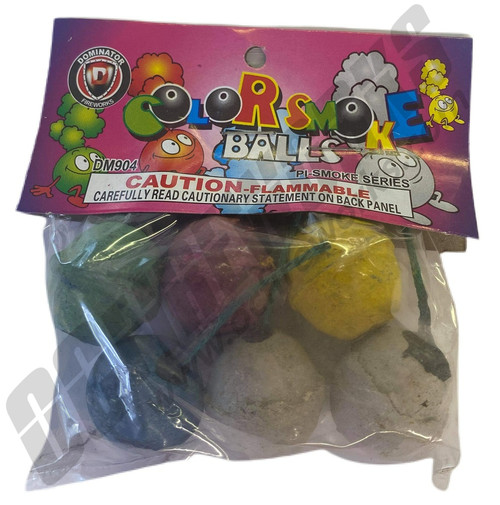The image features a single, centrally positioned package of color smoke balls, enclosed in a transparent plastic bag allowing the viewer to see at least six distinct smoke balls. The visible smoke balls are green, red, yellow, blue, and two that appear white or light-colored. The top section of the package displays the text and logo. The text "Color Smoke Balls" is prominently presented, with the "O"s stylized as spherical shapes. This section also includes a warning that states, "Caution, flammable, carefully read cautionary statement on back panel." Additionally, there are cartoon illustrations of smoke balls with smiling faces and colored puffs coming from their heads, such as a green smoke ball with a green puff located in the bottom left corner. The top left of the packaging features the Dominator Fireworks logo, emphasizing the brand.